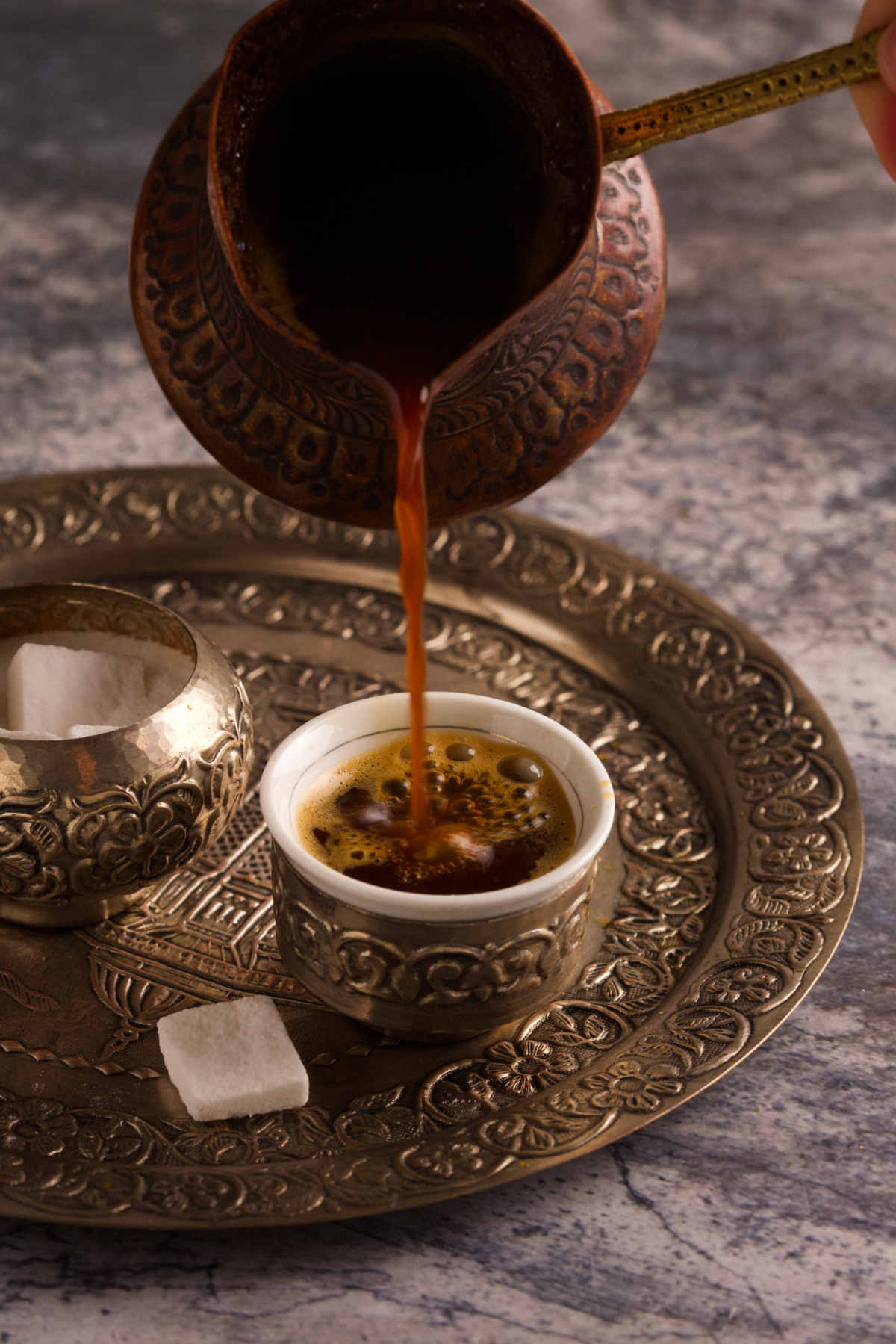This is a detailed color photograph capturing a moment of someone pouring hot, frothy coffee, possibly Turkish coffee or espresso, from an ornate brass pitcher with a long handle and intricate etchings. You can see the edge of the pourer's hand in the upper right corner. The coffee is being poured into a distinctive coffee cup, which has a ceramic interior and a silver or brass exterior, featuring a matching ornate design. The cup is nearly full, with bubbles indicating the warmth and freshness of the coffee. The setting is a luxurious marble tabletop, atop which sits a golden, intricately designed tray. On this tray, there's a matching golden-trimmed plate holding the coffee cup. Alongside the cup, a large cube of sugar rests on the plate. Nearby, a golden sugar bowl containing additional large sugar lumps complements the setup. The overall scene is one of opulence and meticulous design, showcasing the pour and the richness of the moment.